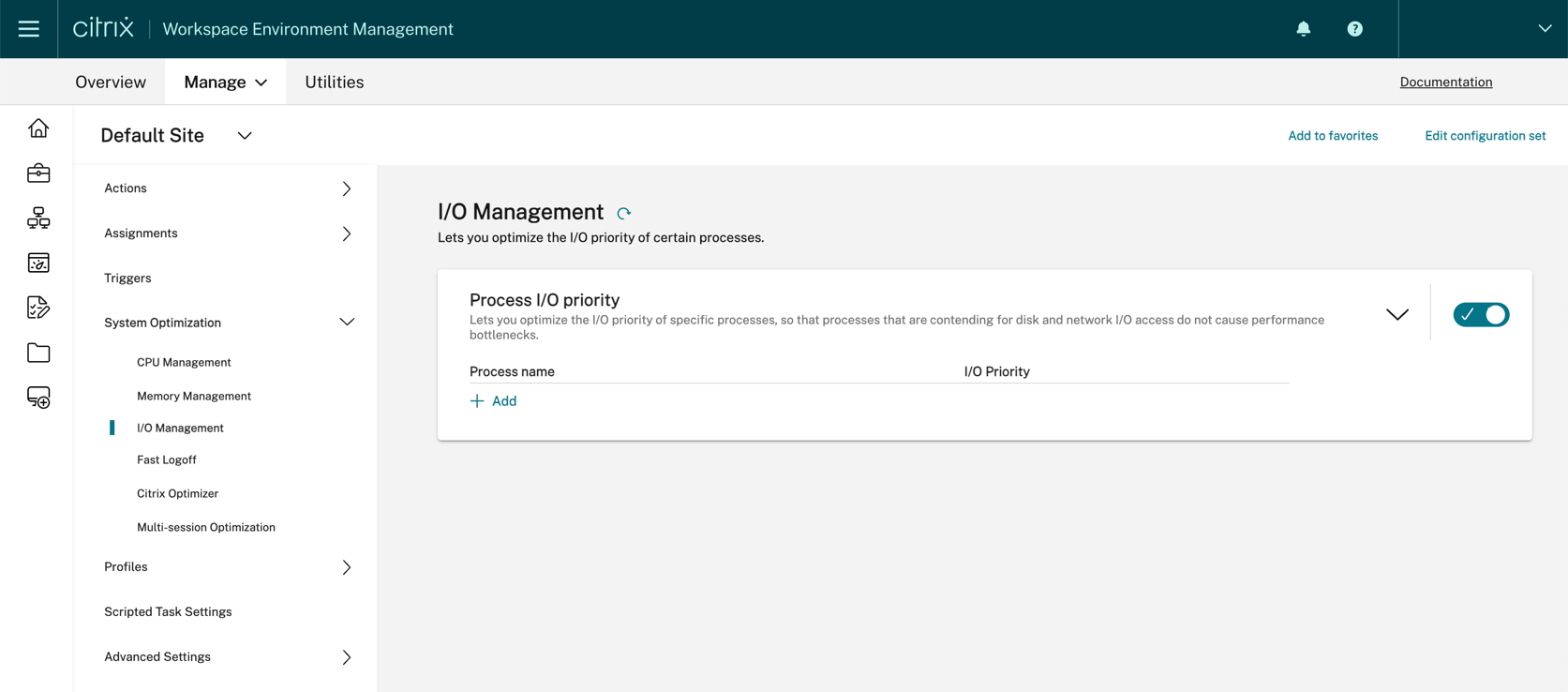The image depicts a webpage interface for Citrix Workspace Environment Management. At the top, there's a dark blue horizontal bar featuring three horizontal lines stacked on top of each other, next to the "CITRIX" logo with a dot above the "X". Beside the logo, separated by a vertical line, is the title "Workspace Environment Management."

Towards the right end of the bar, there is a white bell icon, followed by a solid white bubble containing a grayed-out question mark. Further to the right, there is a downward-pointing "V" shape.

Beneath this top bar, three navigation options are displayed: "Overview," "Manage," and "Utilities," with "Manage" being the current selection. Directly below this, "Default Site" is indicated, and several sub-options are listed: "Actions," "Assignments," "Triggers," "System Optimization," "Profiles," "Scripted Task Settings," and "Advanced Settings." The "System Optimization" option has been selected.

Under "System Optimization," the subcategories include "CPU Management," "Memory Management," "I/O Management," "Fast Logoff," "Citrix Optimizer," and "Multi-Session Optimization." "I/O Management" is highlighted, with a brief description stating, "Let you optimize the I/O priority of certain processes." Below this, a white box labeled "Process I/O Priority" contains gray writing that explains, "Let you optimize the I/O priority of specific processes so that they are contending for disk and network I/O access. Do not cause performance bottlenecks."

Beneath this, there is a dark teal bubble with a downward-pointing "V" on the right and a white check mark on the left, followed by the label "Process Name" in the middle and "I/O Priority" underlined. At the bottom of the box, a light green "+ Add" button is visible.